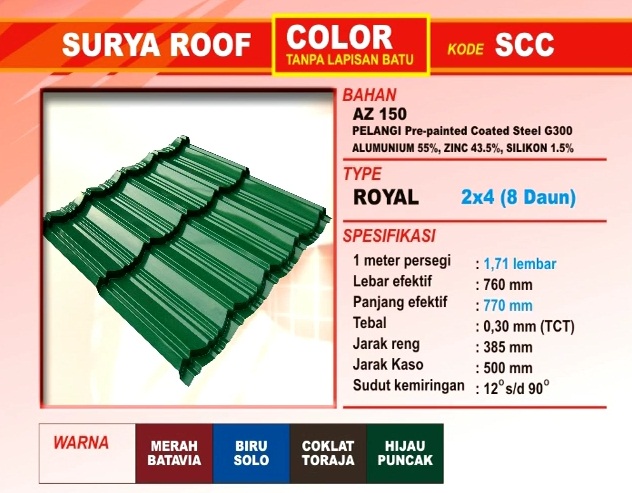The image appears to be a computer-generated listing from a sales catalog or home improvement website, featuring a roofing product. The top of the image has a red banner with orange borders, displaying the text in white letters: "Surya Roof." Adjacent to this is a yellow rectangle containing the text "Color Tanpu Lapisan Batu" and the code "SCC." Below this header, on the left side, there's a visual of green roof shingles with ridges that resemble hard plastic or coated steel. The background behind the image features a pinkish-salmon border. To the right of the shingle image is a detailed description set against a pink background, in black font, listing the material as "Pelangi Pre-Painted Coated Steel G300 Aluminum Zinc Silicon" and mentioning the specifications such as "Bahan AZ 150 type Royal 2x4." The colors present in the image include pink, red, orange, yellow, green, brown, white, and black.